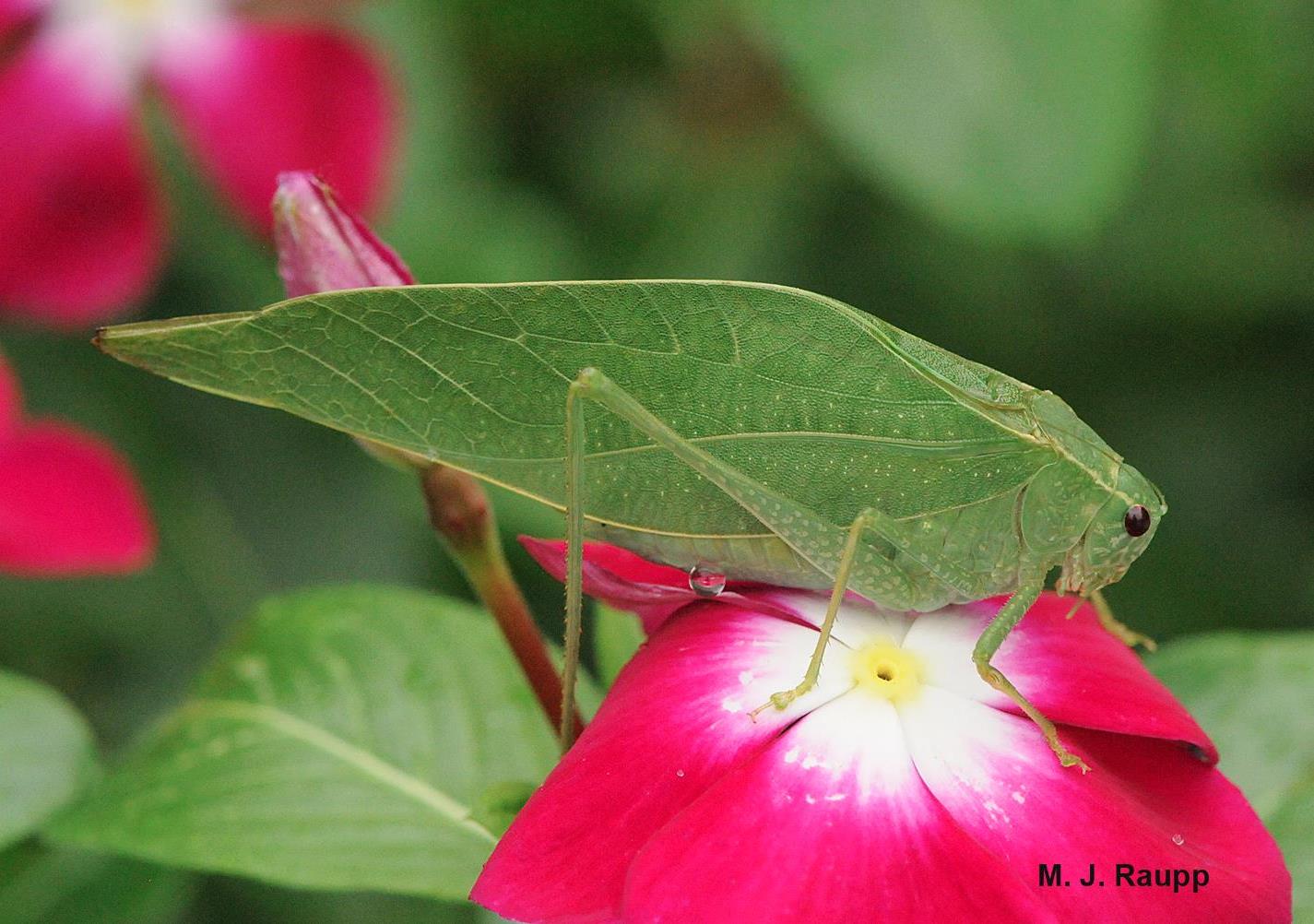This image is a highly detailed close-up of a green insect, perfectly camouflaged to resemble a leaf. The insect is perched on a vibrant magenta flower, which fades to white as it nears the stem, and features a creamy white center with a hint of yellow. The background is filled with blurry leaves and more of the same magenta flowers, adding depth to the scene. The bug’s head is positioned to the right center of the image, with its body extending towards the left. You can clearly see three of its slender legs adorned with yellow spots and tiny barbs. It has a textured, veined, light green body that mimics a leaf and a single large, dark eye. A dewdrop clings to its abdomen, adding a touch of realism. The name "MJ Raupp," likely the photographer, is displayed in the bottom right corner.